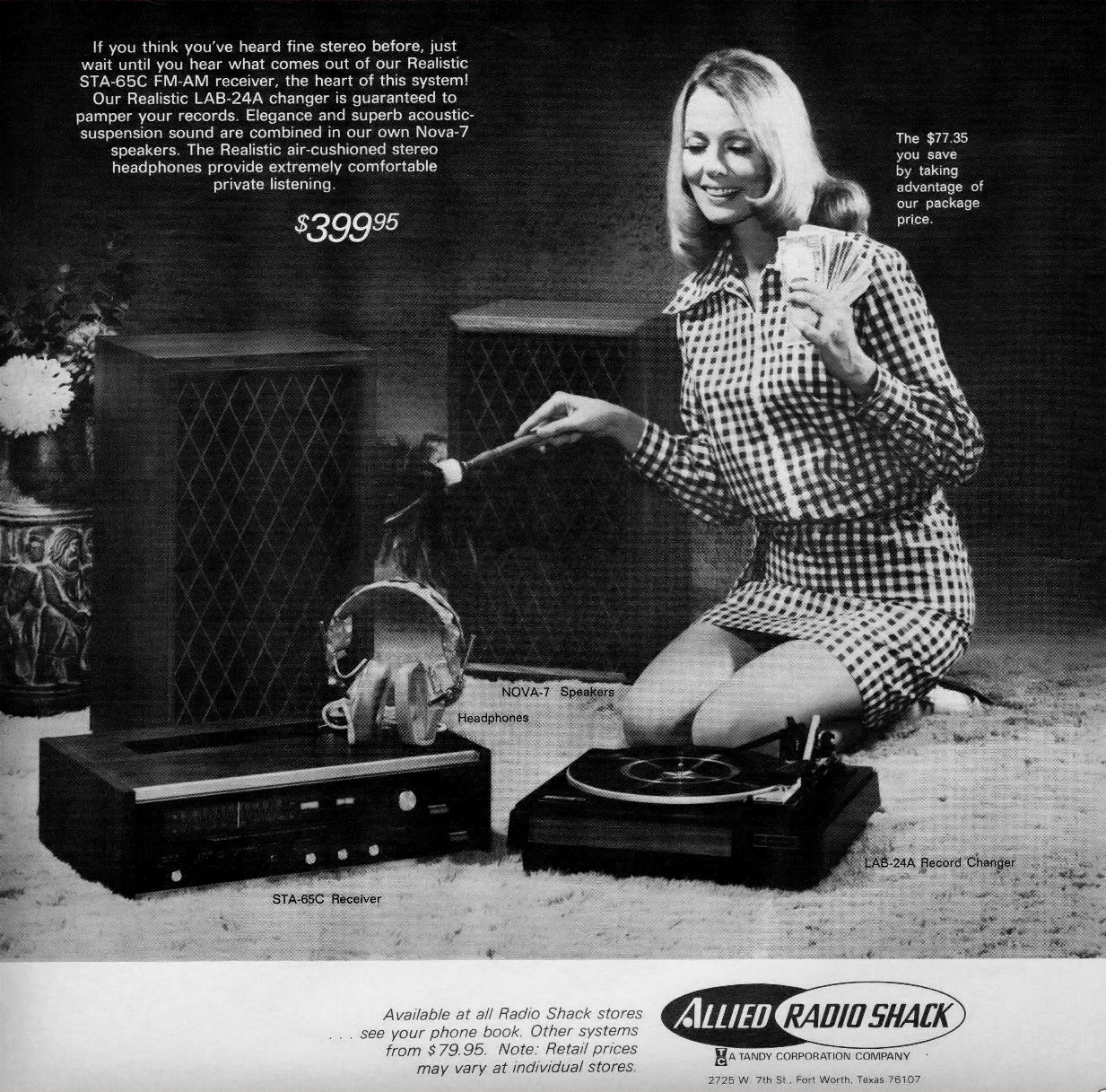This vintage black-and-white advertisement from the 1960s or 1950s promotes various audio equipment sold at Radio Shack. The image features a woman with a flip-style haircut, dressed in a checkered, tattered top, kneeling on a rug. In her right hand, she holds a bunch of money, while her left hand extends a roasting stick with a marshmallow, adding a whimsical touch to the scene. Surrounding her are essential audio devices: a large speaker with a diamond-pattern grill, a vintage sound system, a record turntable, and a pair of stereo headphones. Another identical speaker stands behind her, enhancing the display. The text highlights the featured products, including the Realistic STA-65C FM AM receiver, the LAB-24A record changer, and Nova 7 speakers, all promising elegance and superb sound quality. The accompanying realistic air-cushioned stereo headphones promise comfort for private listening. Priced at $399.95, the ad claims a savings of $77.35 with the package and urges customers to visit Radio Shack stores, as noted in a white rectangle at the bottom. The Allied Radio Shack logo marks the bottom corner, cementing the advertisement’s vintage credibility.